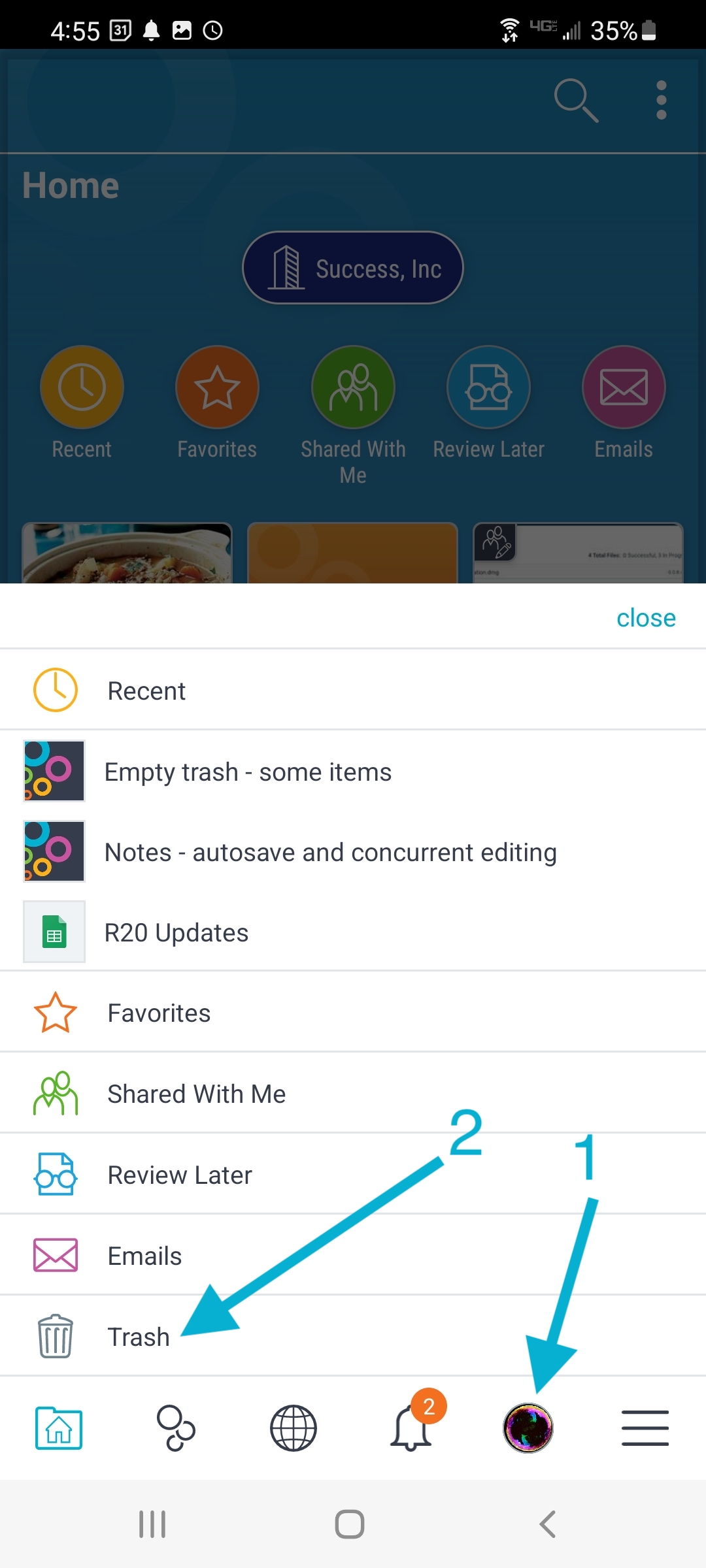A detailed and cleaned-up description of the image:

---

The image is a screenshot captured from a smartphone displaying an interface that appears to be part of an application. The status indicators at the top of the screen confirm it's a smartphone; the time is shown as 4:55 on the top left, and the battery level is indicated at 35% on the top right. The majority of the screen has a dark background, contrasting sharply with a bright white popup window at the bottom.

The white popup window is a user interface menu titled "Recent". Within this menu, a list of options is provided, including "Empty Trash," "Some Items," "Notes," "Auto-save," and "Concurrent Editing." Further down, additional menu options are displayed: "R20 Updates," "Favorites," "Shared with Me," "Review Later," "Emails," and "Trash."

Two blue arrows within the popup section are annotated with the numbers "1" and "2". Arrow number "1" is pointing to a small black symbol toward the bottom of the screen, while arrow number "2" directs attention towards the "Trash" option. The purpose of these arrows isn't clearly explained, but they may be intended to guide users on how to move items to the trash, possibly suggesting a drag-and-drop interaction.

Additionally, a notification bell icon is situated within this interface, indicating that there are two unread notifications for the user.

---

This description thoroughly details the visual aspects and probable functionality of the screenshot, aiding in a clear understanding of the image content.